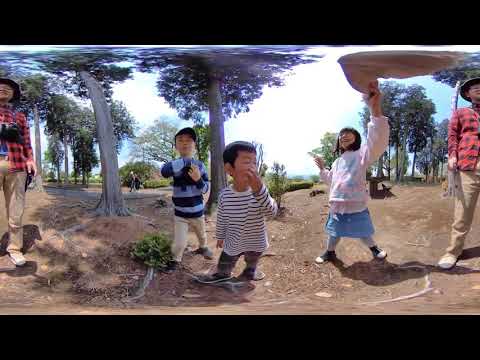The slightly out-of-focus, full-color photograph captures an Asian family outdoors during the daytime in a setting resembling a park, with mostly brown dirt and some scattered rocks and vegetation. The image is horizontally rectangular with black borders only on the top and bottom. In the background, there are green-leaved trees and shorter shrubs. Depicted are two adults and three young children. On the far right stands a gentleman in chinos, a red plaid shirt, and a hat. Next to him is a little girl in a pink top and blue skirt, raising something above her head. In the middle are two boys, both in striped shirts—one with smaller, black and white stripes covering his laugh, and the other, with larger stripes, wearing chinos and a hat while gesturing with his hands. To the far left is a woman, possibly the mother, dressed similarly to the man in chinos, a plaid shirt, and a hat, holding a camera.